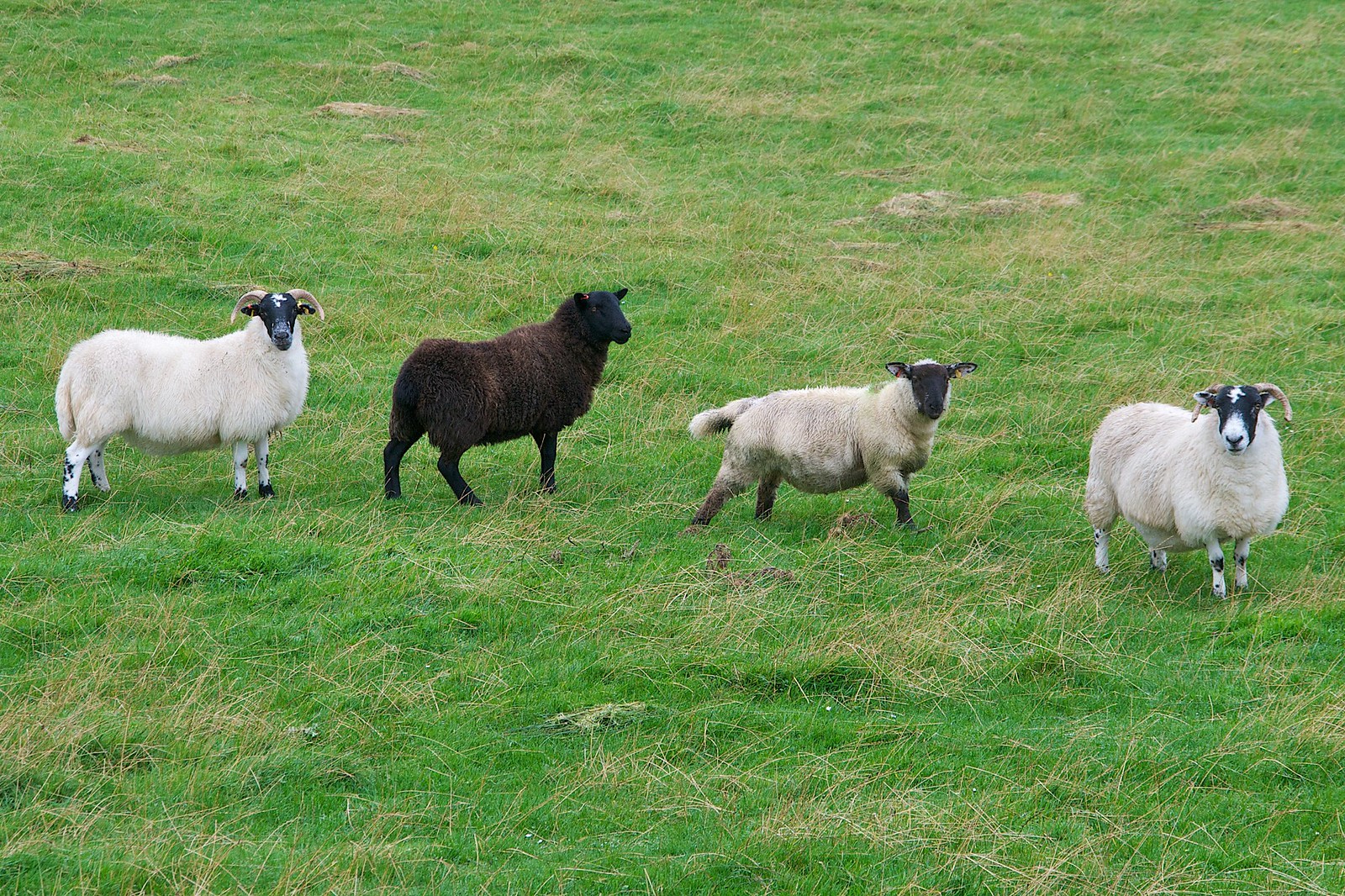The photograph captures an outdoor scene of a lush green meadow interspersed with light brown reeds and patches of hay, presenting a serene, semi-professional quality image. The image, centered on four sheep standing in a slight line on a gentle hill, is devoid of any other objects or elements, allowing full focus on the animals and their natural surroundings. From left to right, the first sheep is a pristine white with black face and legs, and distinctive horns that curve downwards, featuring a white tuft on its head. Next to it stands a completely black sheep, including black legs, ears, and face, with its back half-turned away from the camera. The third sheep displays a dirtier, beige coat with black feet and face. The line ends with another white sheep, mirroring the first’s features, with black and white legs, a black and white face that creates a masked appearance, and downward curving horns. The sheep are aligned almost horizontally with three of them gazing towards the camera, while one, slightly turned, looks back, adding a sense of curiosity to the composition.